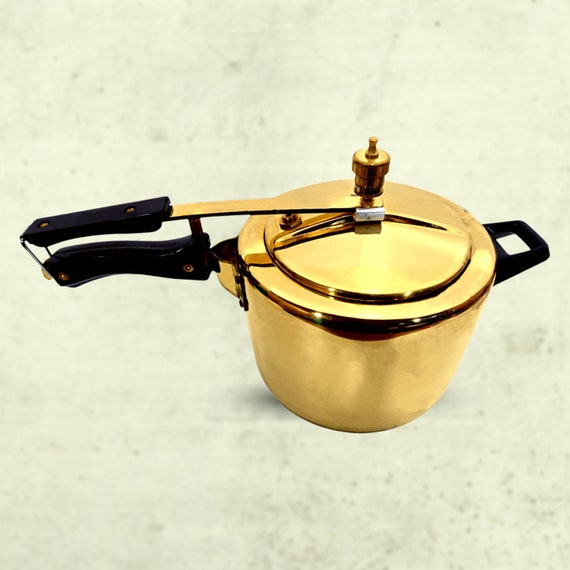The image depicts a retro-style kitchen scene featuring a distinctive and ornate golden pot, which resembles a pressure cooker, sitting on a white speckled stone or possibly granite countertop. The pot itself is a bright gold color, including its permanently attached lid, which adds to its unique appearance. At the top of the lid, there is a mechanism resembling a dial or thumb screw that appears to be part of a locking system. 

The pot has two black handles: one on the side for holding, and another connected via a metal pin designed to lift the lid when squeezed. The intricate design of the pot, with its combination of golden color and black handles, adds a striking contrast to the kitchen's retro aesthetic. The muted pale green or white background further enhances the vintage vibe, making the pot a focal point in this charming kitchen setting.